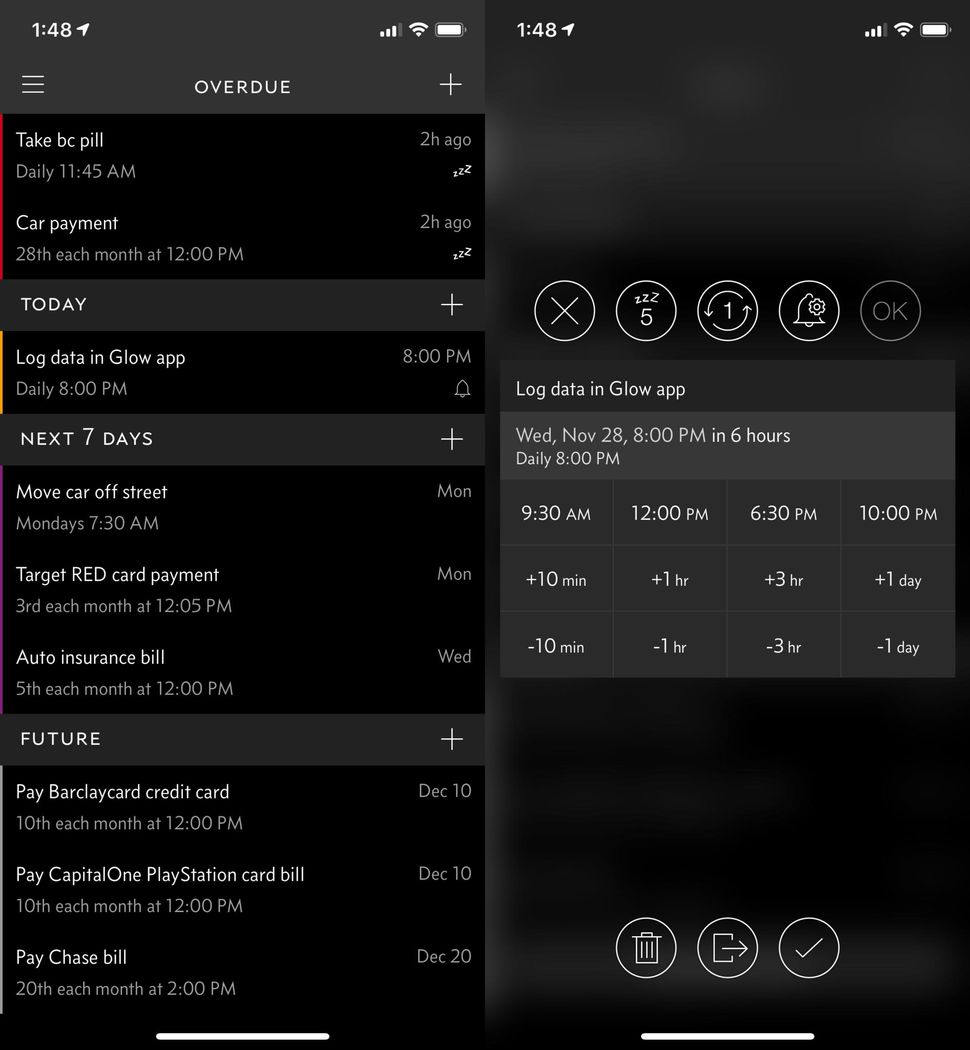The image depicts a highly detailed and wide dual-screen display, possibly on a tablet or a foldable phone, with a sleek dark charcoal color. Both screens show identical times, 1:48, and indicate full battery power.

### Left Screen:
The left screen features a "To-Do" list labeled "Overdue". It includes a hamburger menu icon on the top left, followed by a series of overdue tasks:
- **Take BC Pill**: Due two hours ago.
- **Car Payment**: Due two hours ago.
- **Log Data in the Glow App**: Scheduled for 8 p.m. today, with a reminder to log data daily at 8 a.m.
- **Move Car Off Street**: Scheduled for Monday at 7:30 a.m.
- **Target Red Card Payment**: Due the 3rd of each month at 2:05 p.m.
- **Auto Insurance Bill**: Due at 12 p.m.
- **Future Tasks**:
    - **Pay Barclay Credit Card**: Due on the 10th.
    - **Pay Capital One Bill**: Due on the 10th.
    - **Pay PlayStation Card Bill**: Due on the 10th.
    - **Pay Chase Bill**: Due on the 20th at 2 p.m.

It is evident from this list that the individual is behind on a number of payments and tasks.

### Right Screen:
The right screen seems to depict an attempt to log data into the "Glow App", likely related to the previously mentioned overdue task. There's a clear emphasis on the user's urgent need to manage and complete these tasks to avoid further delays.

Overall, the image conveys a sense of urgency for the individual to catch up on numerous overdue payments and tasks, emphasizing the importance of timely completion and organization.